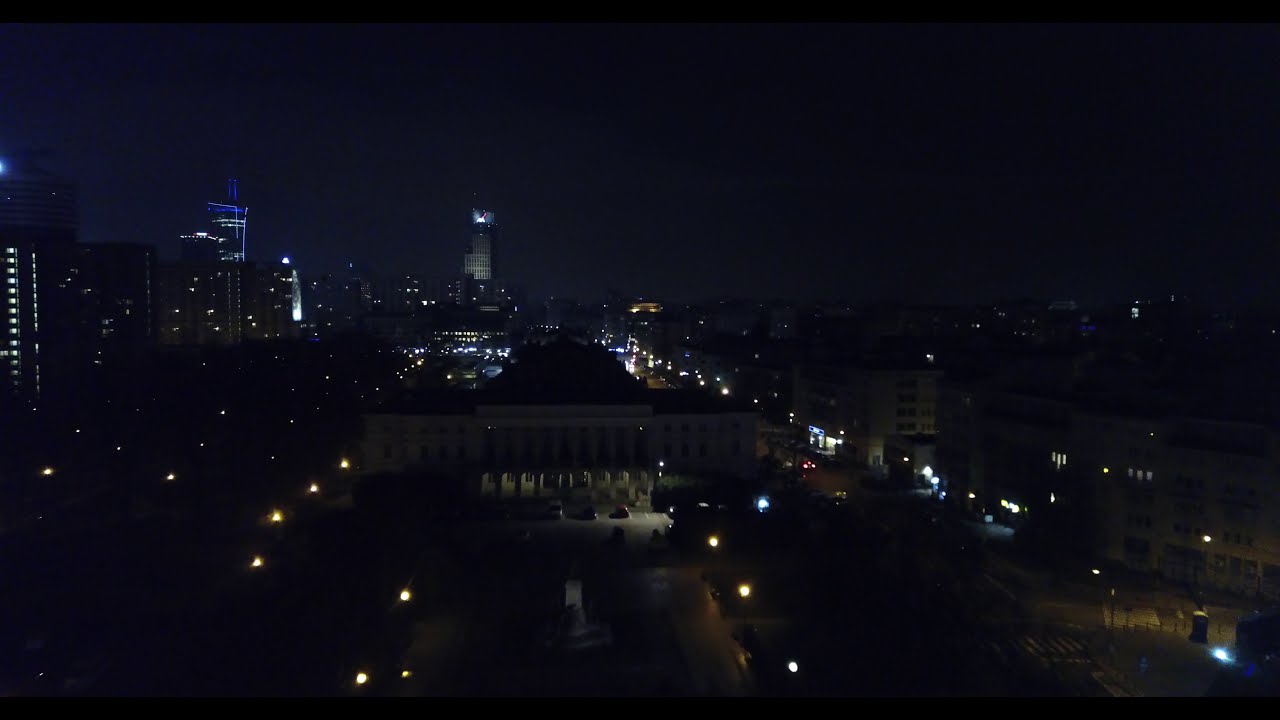The image depicts a nighttime cityscape with a striking skyline dominated by tall buildings illuminated by various colored lights. In the distance, several tall buildings stand prominently, including one with white lights at the top and another with blue lights. These are flanked by additional smaller buildings dotted with lights in their windows. In the center of the image, a shorter, distinguished building with a dark, dome-like roof and numerous pillars at its forefront captures attention. This building is reminiscent of a government structure and is surrounded by lights lining a reflective water pool with a fountain in its middle. The right side of the image features shorter buildings, well-lit streets, and streetlights casting a soft yellow glow, suggesting a bustling thoroughfare below. The photograph was taken from an elevated vantage point, offering a comprehensive yet moody view of the city under the cloak of night.